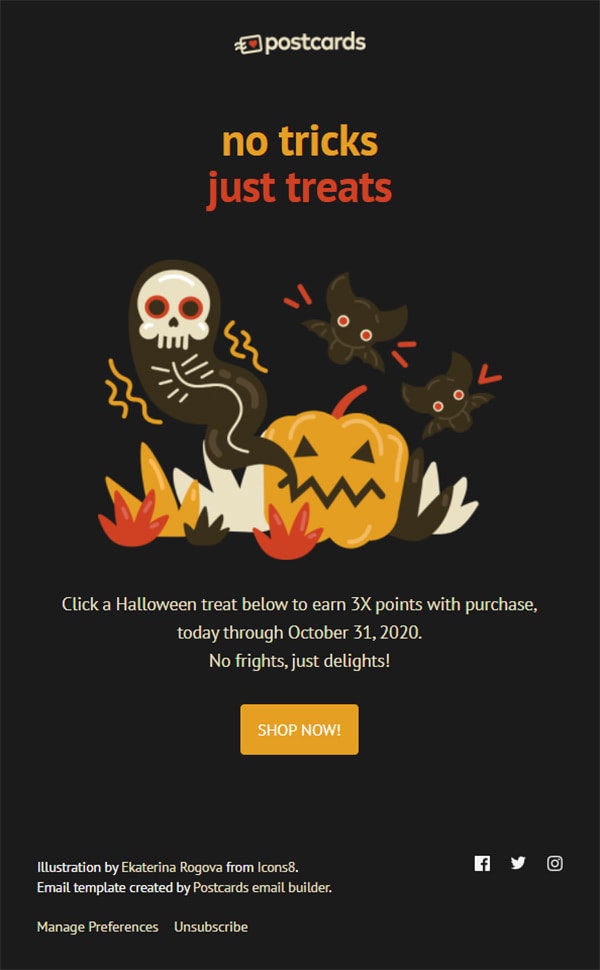Here is a cleaned-up and detailed caption based on the provided description:

---

The image appears to be a screen capture of marketing material for a company named Postcards, featuring a predominantly black background. At the very top center, the company's logo and name, "Postcards," are displayed. Positioned directly beneath this is the phrase "No Tricks" in a burnt yellow color, followed by "Just Treats" written in a reddish hue.

Taking center stage in the graphic is a festive Halloween scene, featuring a jack-o'-lantern flanked by two cartoonish bats in flight. To the left of the pumpkin, a ghostly figure reveals a partial skeleton with a skull and ribcage. Surrounding these central elements are decorative graphics resembling leaves.

Accompanying this visual is an enticing message: "Click a Halloween treat below to earn three times points with purchase today through October 31st, 2020. No Frights, Just Delights." Just below this message, a prominent "Shop Now" button invites immediate action.

In the bottom left-hand corner, small white text credits the illustration to Ekaterina Rogova from Icons 8, notes that the email template was created by the Postcards email builder, and includes links for managing preferences and unsubscribing. The bottom right-hand corner features hyperlinks to the company's social media profiles on Facebook, Twitter, and Instagram.